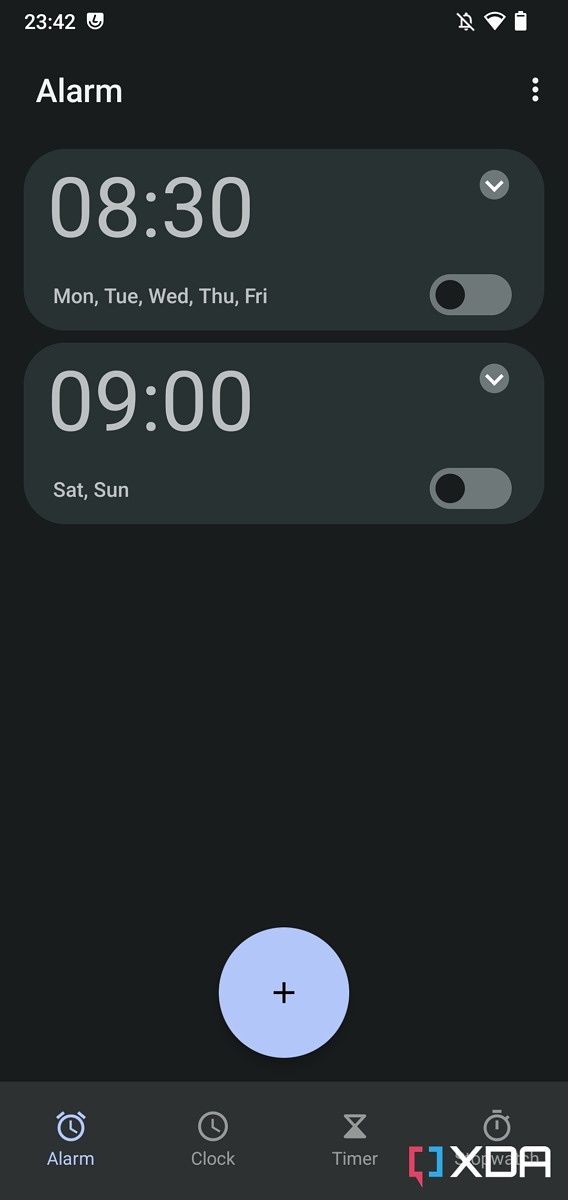The image is a screenshot of a mobile device displaying an alarm or clock app. The device's interface (UI) is visible at the top, featuring the time set to 23:42 in military format. To the right of the time is an icon that resembles a semicircle with a nose and a smile, though the specific app it represents is unclear. Additionally, three other icons are visible: a silent mode icon indicating notifications are muted, a Wi-Fi symbol, and a battery indicator showing approximately 80-90% charge without a percentage value.

The main part of the screen showcases the alarm settings. At the top, a header labeled "Alarm" is displayed. Below it, two alarms are listed but are not activated. The first alarm is set for 08:30 on weekdays (Monday through Friday), and the second is set for 09:00 on weekends (Saturday and Sunday). Both alarms have their toggles switched off.

Beneath the alarm list is a large blue button with a plus symbol for adding additional alarms. The bottom portion of the screen contains a navigation tab with options labeled "Alarm," "Clock," "Timer," and a partially obscured "Stopwatch." A watermark reading “XDA” is visible on the bottom right, partially obstructing the view. The app's color scheme primarily consists of gray tones with light blue accents.